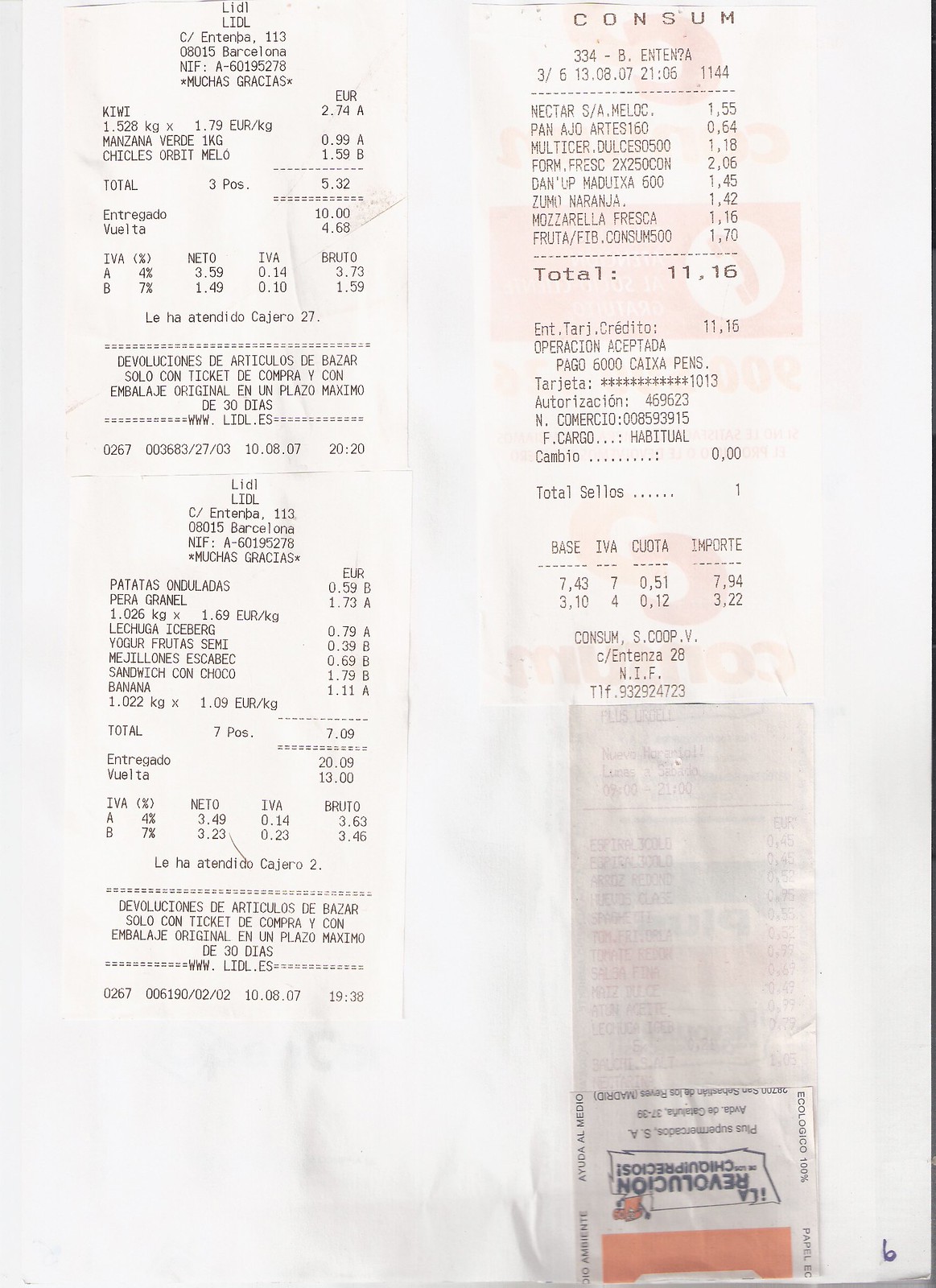The photograph features a collection of receipts set against a white background, all printed on white paper with black text. The two receipts on the left are plain white and originate from Lidl in Barcelona, identifiable by their address information. Lidl appears to be a grocery store as the listed items include iceberg lettuce, a sandwich, and kiwis. The text on these receipts is predominantly in Spanish, although some English words are discernible.

The receipt on the right stands out due to a very light orange watermark and is from a location called Consume. Beneath this receipt, a slightly darker receipt appears, showing the back side. The specific items purchased at Consume are not clear, but they seem to be food-related as well.